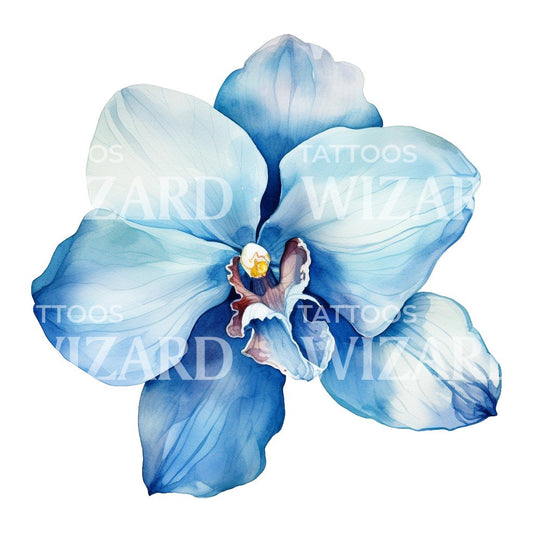This image showcases a close-up of a watercolor painting of a blue flower set against a stark white background. The flower features six prominent, large, wavy petals that range in shades from light blue to dark blue, with hints of white. These petals are asymmetrically arranged, creating a denser cluster towards the top of the image, while the bottom appears to have a missing petal, with a curled one taking its place. The center of the flower is a yellow, almost round structure, reminiscent of a pistil, that gives the appearance of a small, yellow-white flower itself. Additionally, there is a blue petal beneath the yellow center that is tinged with reddish-brown near its middle. Overlaying the image are four semi-opaque white watermarks reading "Tattoos Wizard," with two near the top and two near the bottom, blending into the lighter parts of the flower and background, making them more difficult to discern in those areas.